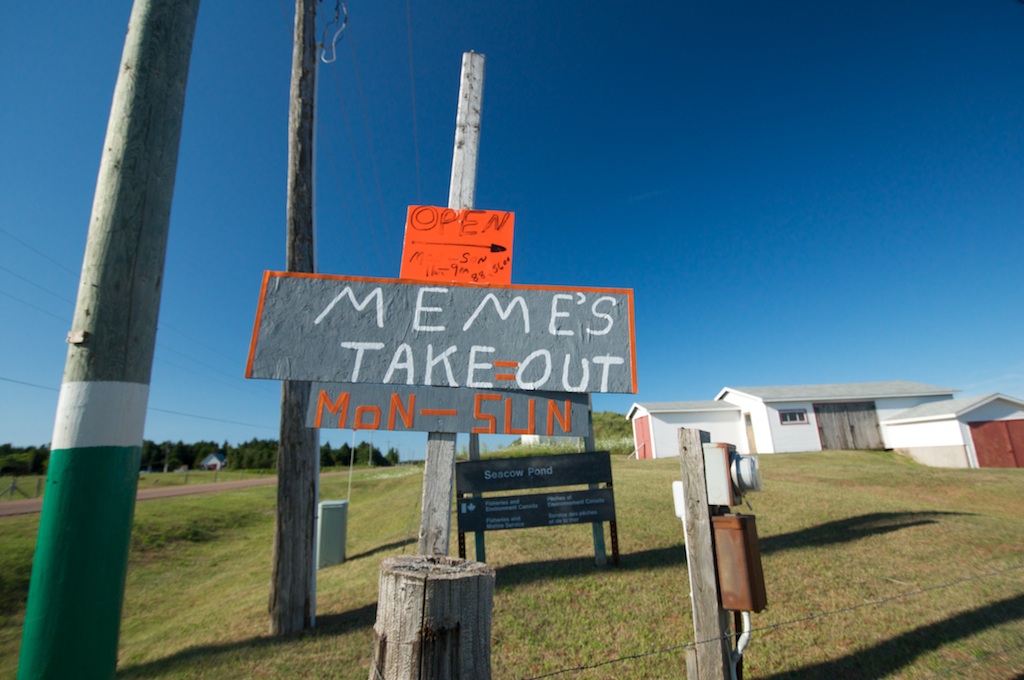This photograph captures a rural, seemingly remote setting. Central to the image is a rustic, hand-painted sign, grey in color with white text that reads "Memes Take Out." Below, the days of operation, "Monday through Sunday," are highlighted in orange. An eye-catching fluorescent orange sticker affixed to the top of the sign announces "OPEN" in handwritten letters, with an arrow pointing presumably towards the location of the takeout service. The sign is mounted on what appears to be a wooden pole, surrounded by additional utility poles, reminiscent of telephone poles.

Adjacent to this setup is an official green sign embedded into the ground, which labels the area as "Sea Cow Pond." The signs and poles stand on a well-kept, short green lawn. In the background, there's a modest, single-story white house with a grey roof, typical of rural architecture. A solitary road meanders to the left of the frame, further emphasizing the isolation of the scene. This photograph encapsulates the simplicity and charm of countryside life, with minimal built elements and a focus on the handmade and functional.